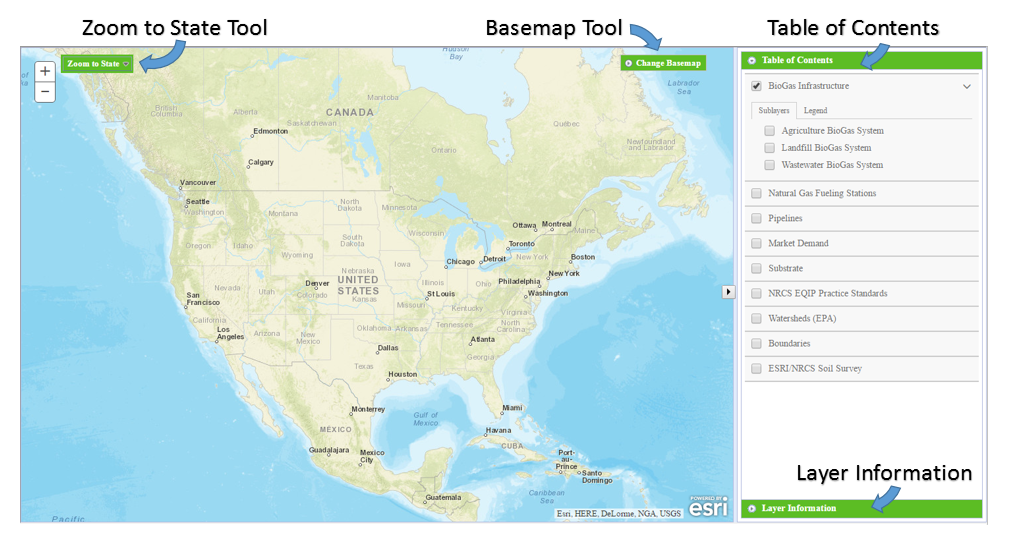This image features a detailed Geographic Information System (GIS) interface displaying a map of the United States, which notably excludes Alaska and Hawaii, but includes Canada. The interface highlights four main tools, each explained with blue arrows pointing to their corresponding green boxes that provide further instructions:

1. **Zoom to State Tool**: An arrow directs attention to a green box labeled "Zoom to State," indicating where users can focus on individual states within the map.
   
2. **Base Map Tool**: Another arrow guides users towards a green box labeled "Change Base Map," suggesting options for altering the visual presentation of the map's base layer.
   
3. **Table of Contents**: Here, an arrow points to a section titled "Table of Contents," which is currently expanded to display "Biogas Infrastructure," illustrating the layers of information that users can explore or toggle.
   
4. **Layer Information**: Lastly, an arrow leads to a green box labeled "Layer Information," indicating where users can find detailed data about the selected map layers.

These components collectively enhance the user's ability to navigate and customize the GIS map interface, making it a versatile tool for visualizing spatial information.